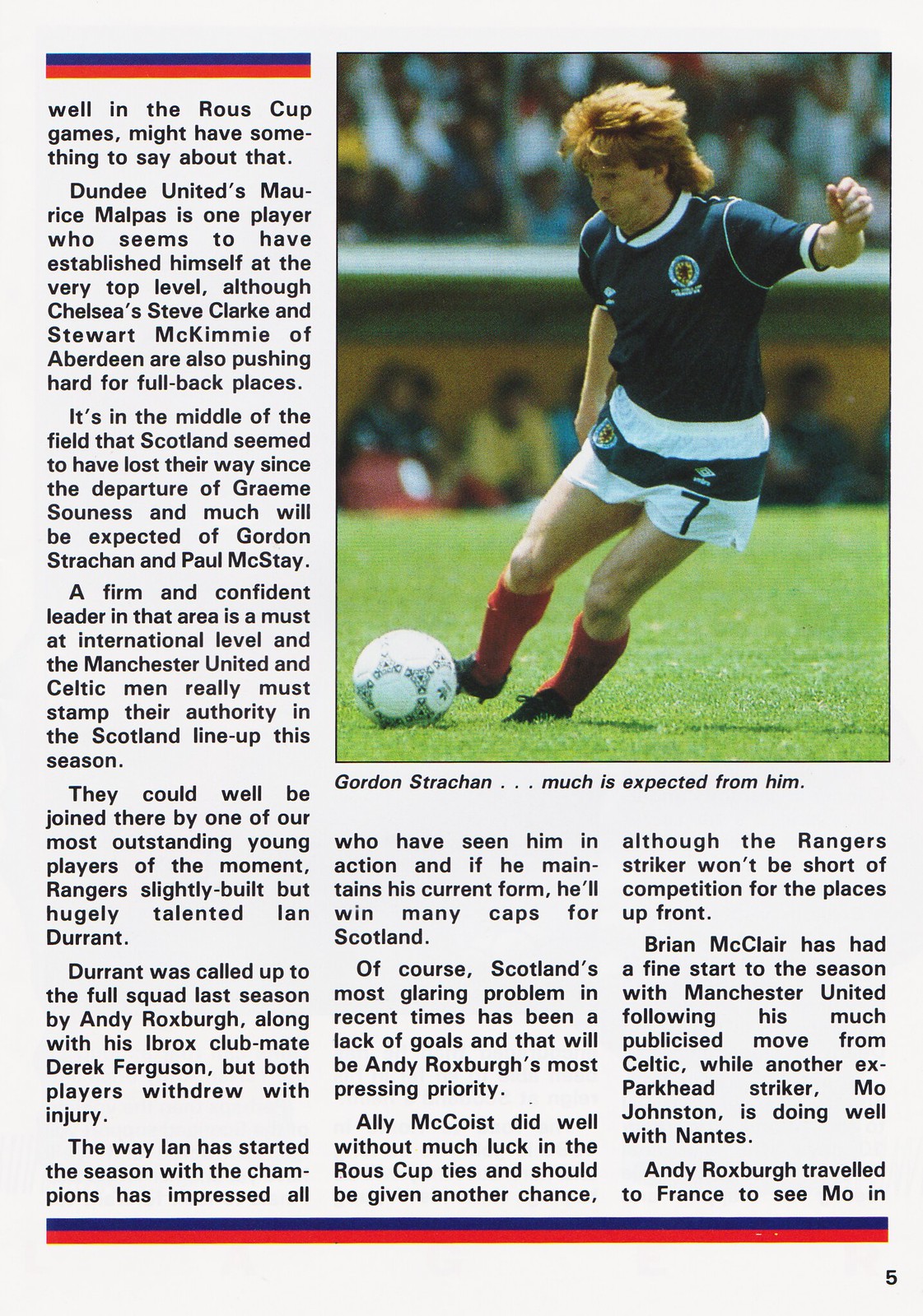The image is a color cutout from a magazine article dating from the 1980s or 1990s. It features a prominent rectangular photo dominating the upper right corner, depicting a man in action. The man, with an orange mullet, is playing soccer and is poised to kick a ball in front of him. He wears a blue short-sleeved jersey paired with white shorts marked with a blue stripe and the number 7. His socks are red. The man appears to be exerting effort, perhaps puffing his cheeks.

In the background, there are blurred spectators, indicating a live soccer match. Above and below the image, there are horizontal blue and red lines. At the bottom right corner, the number 5 is visible. Beneath the photo, the caption reads: "Gordon Strachan, much is expected from him." The accompanying article spans three columns of black text on a white background, discussing Scotland's soccer scene, particularly emphasizing the pressure on Gordon Strachan and Paul McStain to fill the void left by Graeme Souness in the team's midfield.